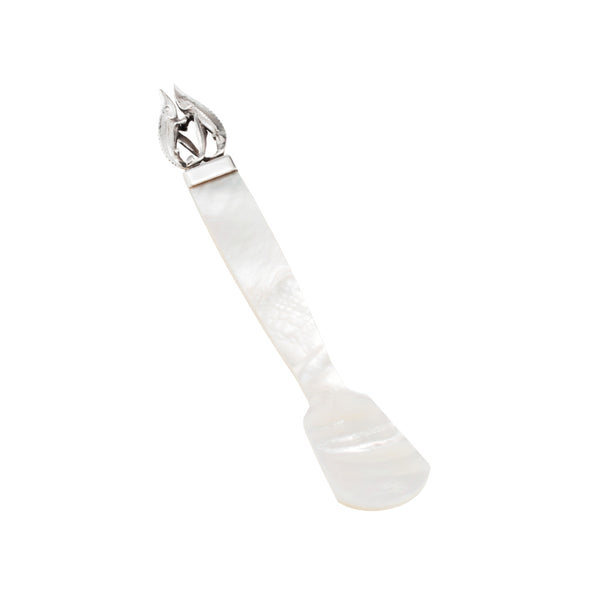The image features an object placed against a solid white background. The object appears to be a utensil with a unique design. The lower half resembles a flat spatula with a white, glossy surface that has a marble-like appearance. The handle is flat and transitions into a metallic portion at the top. This metallic end is elaborately designed, resembling two dolphins jumping in the air, giving it a ribbony, medallion-like look. The combination of these elements creates a piece that is both functional and decorative, though the exact purpose of the object remains unclear.